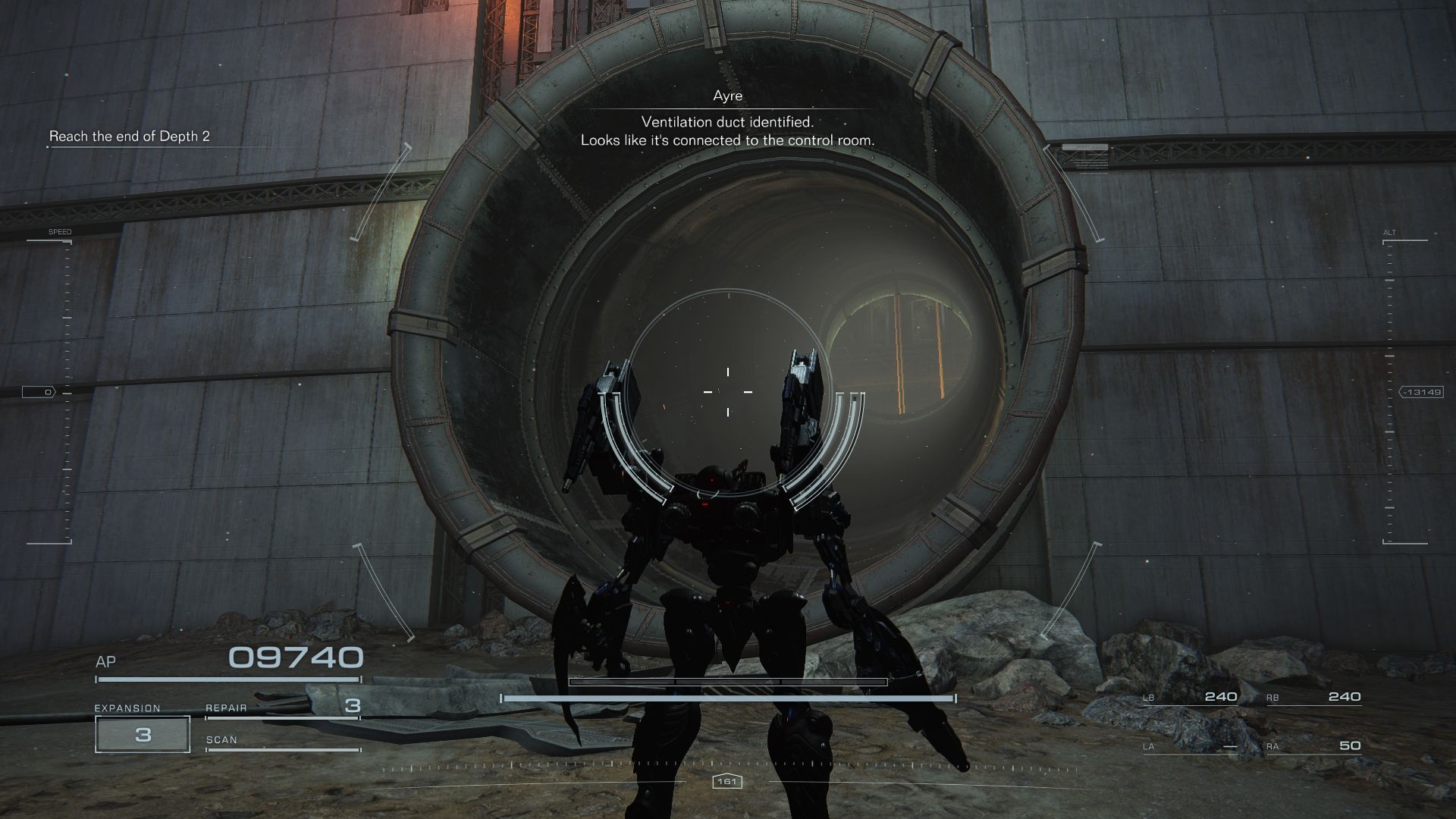The screenshot from the video game displays a detailed environment featuring prominent structures and a unique robotic character. In the center, there's a large circular structure, possibly an air ventilation duct or a sewage tunnel, made of gray concrete with metal bracing two-thirds up its height. The circle has a black rim and glass in the center, resembling a telescope lens, and it's connected to a larger concrete or metal building, potentially a ship. The ground is strewn with rocks, dirt, and rubble.

In the foreground, a headless black robot stands with two arms equipped with what appear to be guns. The robot, seen from a third-person view, has a broad upper body tapering to a thin waist and then widening again into thick legs. Across its frame, the numbers "09740" are displayed, accompanied by some lines. Additionally, a white crosshair in the middle of the image suggests active gameplay, where the robot is interacting with the environment, possibly relaying messages or responding to the objective "reach the end of depth 2." The bottom left corner of the screen shows the character's health or ammunition levels.